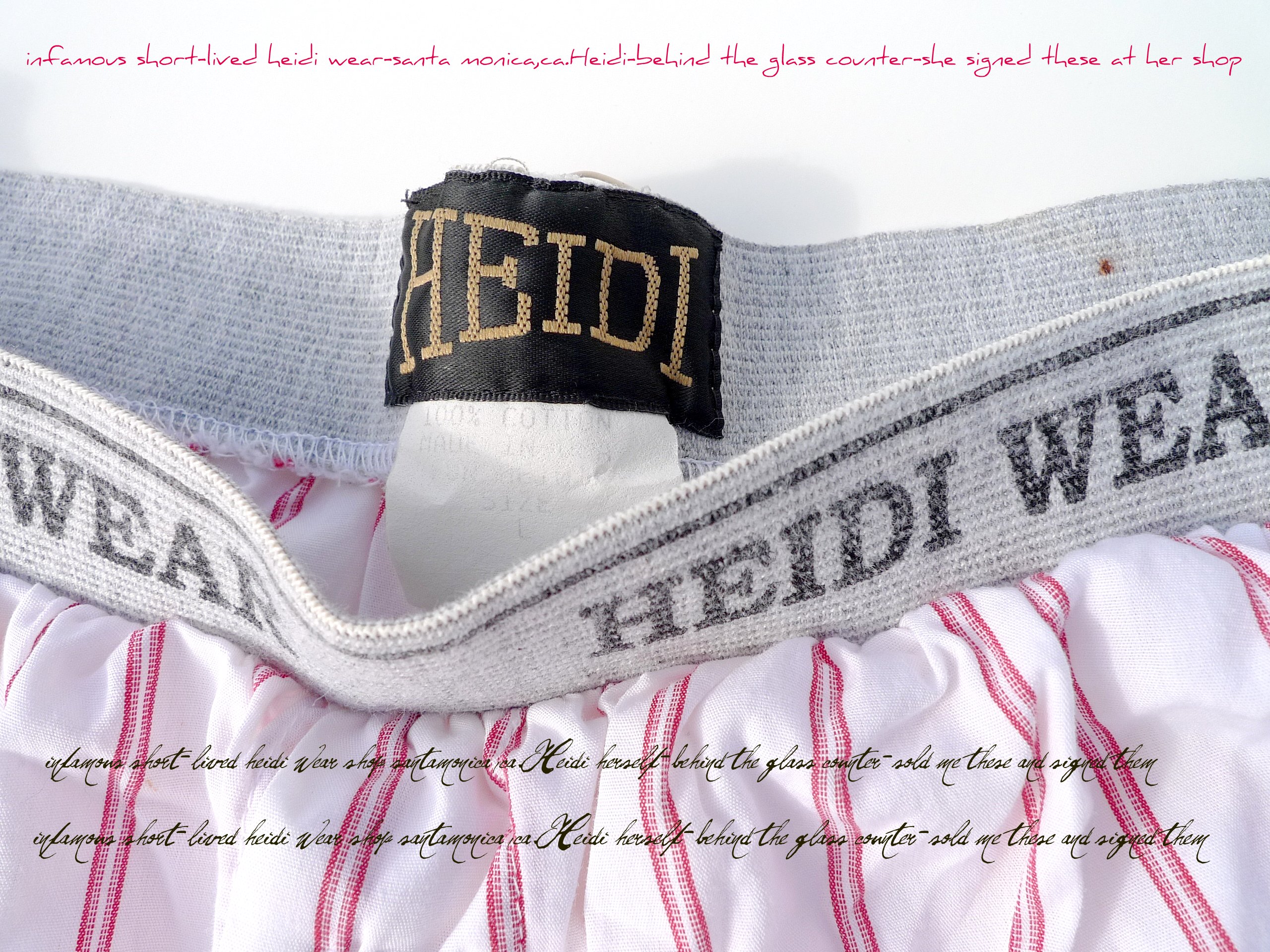This color photograph captures a close-up shot of the infamous short-lived HeidiWear, a brand of underwear from Santa Monica, California. The image prominently features the white elastic waistband, accented with a black line and the black text "HeidiWear." A black label with golden letters spelling "Heidi" is visible on the back of the waistband. Pink letters in a bold font across the top state, "Infamous short-lived HeidiWear, Santa Monica, CA." Below this, it mentions that these items were signed by Heidi herself, who was behind the glass counter at her shop. Although there is cursive black text at the bottom of the photograph, it is too small and difficult to read.